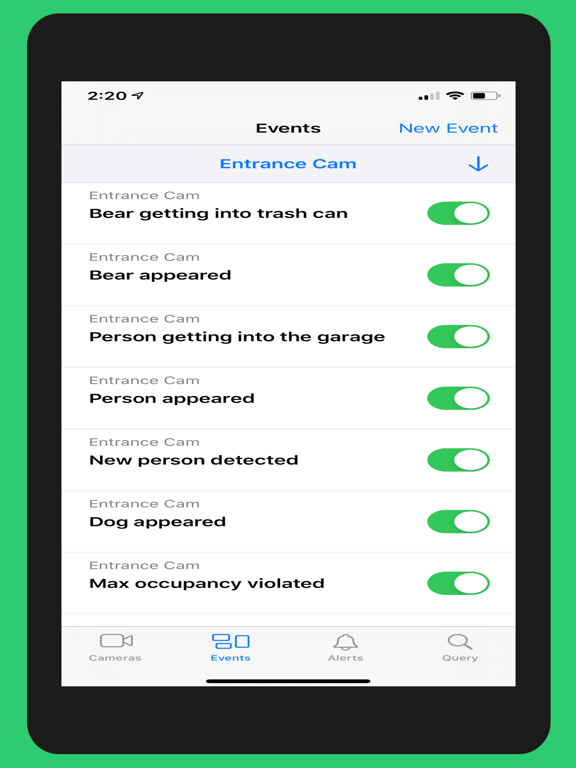The image displays a phone screen with a green-colored message outline. Inside the green box, the time is listed as 2:20. There is a subcategory labeled "Events" in black text. Next to it is the text "New Event" in blue, accompanied by a downward-pointing arrow.

The events include:
- "Entrance Cam: Bear getting into trash can" with a toggled circle symbol indicating it is active.
- "Bear appeared," also with a toggled circle to the right.
- "Person getting into the garage" marked with a white circle to the right.
- "Person appeared" with a similar white circle.
- "New person detected" again with a circle to the right.
- "Dog appeared" with another circle to the right.
- "Max occupancy violated," with the final circle to the right.

At the very bottom of the screen, the categories "Cameras," "Events" (highlighted in blue), and "Query" (spelled out as Q-U-E-R-Y) are listed.